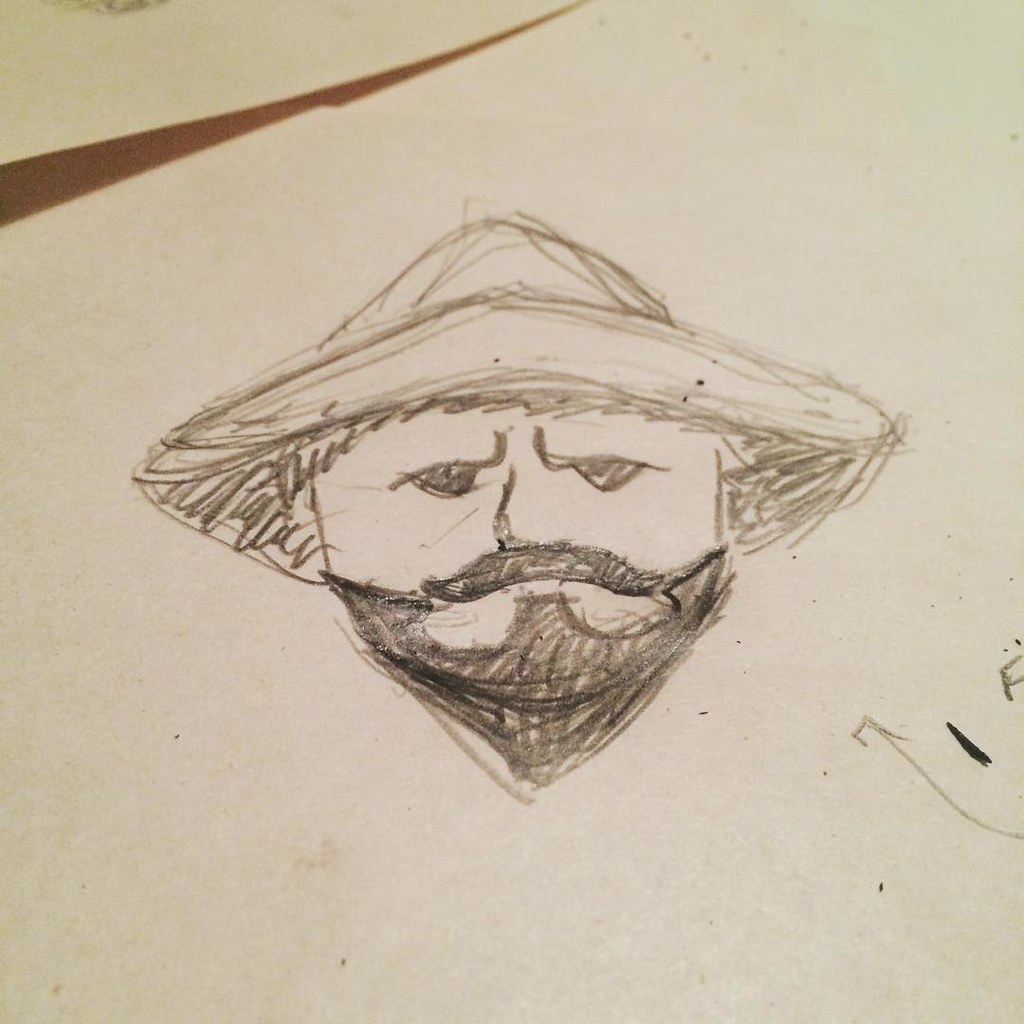In this image, there is a child's drawing of a fisherman. The illustration, amateur in nature, showcases a fisherman wearing a distinctive hat that features a pointed, triangular shape. The fisherman's hat is a notable element, drawing attention with its unusual form. His beard is another prominent feature, colored in with a black felt-tip pen, which contrasts against the rest of the image. The overall drawing appears to be done with a combination of black felt-tip pen and pencil. The composition is quite simple, focusing mainly on the fisherman’s head. Although there are some additional markings on the side of the paper, they do not detract from the central figure. The drawing exudes a whimsical, youthful charm, emphasizing the fisherman's facial features with bold, childlike strokes.